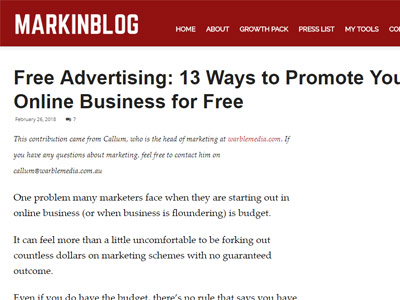Here is the cleaned-up and detailed caption for the given image:

---

Screen capture of a blog titled "Mark in Blog." The header includes navigation links such as "Home," "About," "Growth Pack," "Press," "List," and "My Tools," with more options cut off in the image. The main title of the blog post is "Free Advertising: 13 Ways to Promote Your Online Business for Free," written in italics and slightly difficult to read due to the small font size. A contribution note mentions that the article was written by Callum, the head of marketing at an unspecified website, encouraging readers to contact him at Callum@[samewebsite].com for any marketing questions. The article's introduction discusses the common challenge marketers face concerning budget constraints when starting an online business or when their business is struggling. It highlights the discomfort of spending large sums on uncertain marketing strategies. The text is cut off, leaving the rest of the article unreadable.